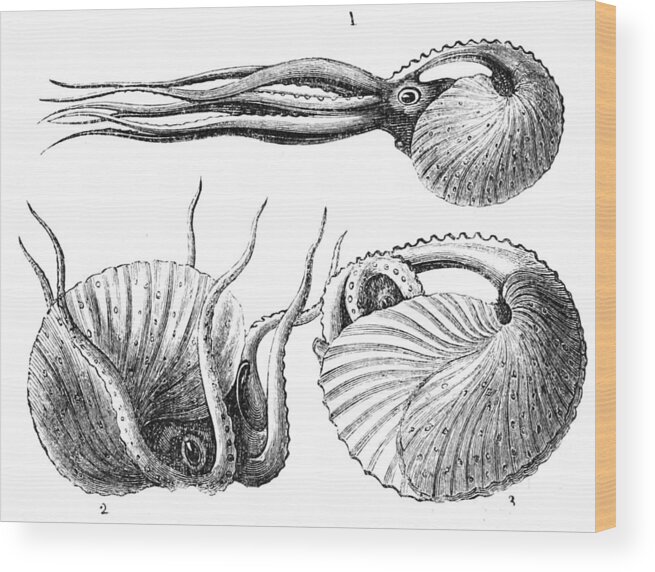The image is a detailed illustration and diagram featuring a hybrid creature resembling both an octopus and a snail, characterized by a series of black and white sketches. The creature, possibly an ancient or fictional species, has an octopus-like body with numerous tentacled arms and a prominent eye, partially encased in a shell-like structure with ridges and spikes. There is an interesting detail of a hole behind the eye, allowing a glimpse through. Depicted in three distinct motions, the first illustration shows the creature swimming horizontally to the right, the second shows it with its tentacles raised as if hanging upside down, and the third depicts it retracting into its shell. All three diagrams are neatly numbered, set against a pale whitish-grey canvas, suggesting the appearance of a purchasable or decorative wooden portrait. The artistic style, combining detailed etching and shading, gives the illustration a unique and almost caricature-like quality.